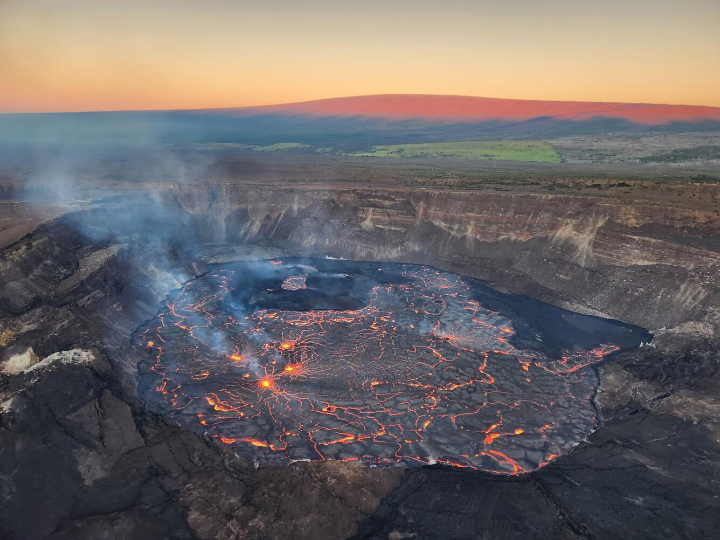The photograph captures an active volcanic caldera during a presumed eruption, with intense geological and thermal activity. Central to the image is a roughly circular, shallow pit, approximately 30 feet in diameter, filled with glowing, molten magma that seeps through cracks in the blackened surface. Rising gray steam and smoke contribute to the evident heat and energy within the caldera. Surrounding this fiery center is a flat, planar landscape cloaked in dark ash and stone, contrasting sharply with the lighter green rolling hills visible in the distance. The sky, tinged with shades of orange, hints at an atmospheric moment of dawn or dusk, casting a dramatic light over the scene. Encircling the caldera are taller rock formations and distant mountainous peaks, their slopes tinged with red from the sunset or sunrise, transitioning to dark tones and ultimately lush green grass further down. The intricate details and stark contrasts within the landscape emphasize the volatile beauty and raw power of the volcanic eruption.